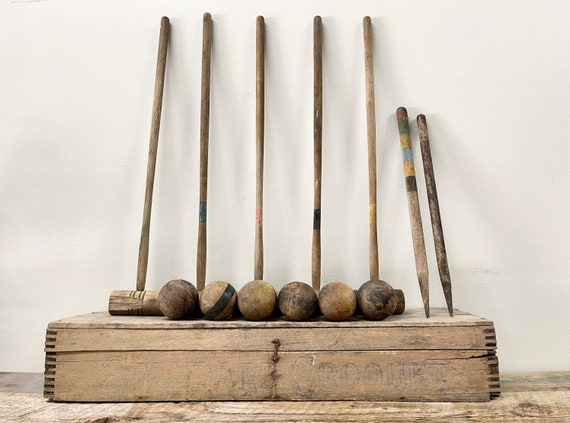This photograph captures a worn, antique croquet set, displayed against a white wall. The set consists of five wooden mallets, six wooden balls, and two stakes, all showing signs of age. The mallets, exhibiting slight inconsistencies in width possibly indicating hand-carving, have their handles leaning against the wall, with the mallet on the left featuring noticeable red stripes on its head. The balls, placed in front of the mallets, include one with a visible black line and others showing faded colors of blue, yellow, brown, green, and white. Two stakes also lean against the wall, one matching the balls' neutral tones, while the other exhibits vibrant yellow, brown, blue, and green elements. All these items rest on an old, closed wooden box, barely revealing the word ‘Croquet’ in faded blue lettering, which is itself placed on a slightly glossy wooden surface.